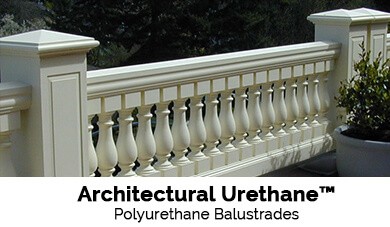This advertisement features a detailed color photograph of a white railing, likely used for balconies, terraces, or bridges in elaborate and expensive homes. The railing is made from an architectural urethane material, specifically polyurethane balustrades, as noted by the line of text at the bottom of the image reading "Architectural Urethane™ Polyurethane Balustrades." The railing is composed of horizontal support elements at the top and bottom, connecting approximately 15 to 17 spindle-like balusters in the middle, which are shaped for a decorative effect, resembling bowling pins. A vertical support column anchors the balustrades. The scene past the railing includes a variety of green, white, black, and possibly gray trees, with a plant and planter situated to the right of the railing. This innovative material aims to replicate the traditional look of stone or wood railings commonly found in European architecture, but with modern advancements.